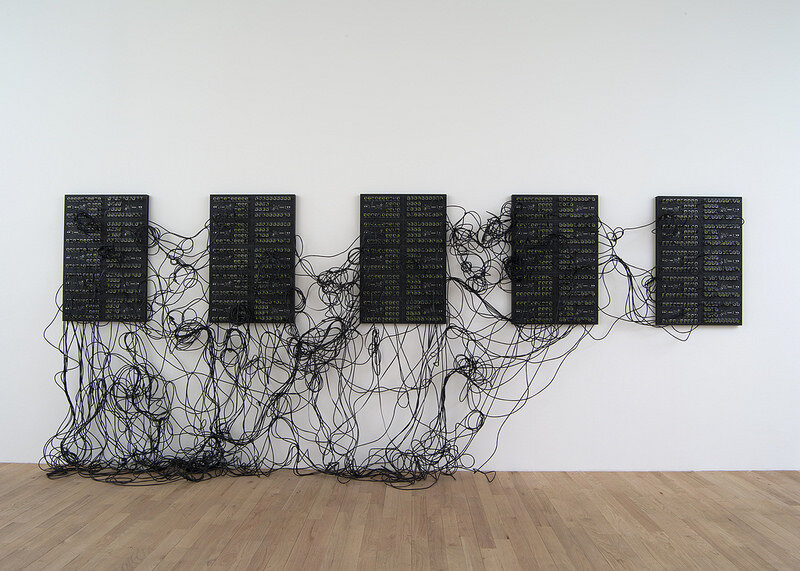The photograph captures an indoor setting with a white wall as the backdrop. Prominently displayed on the wall is a series of five black circuit boards arranged in a neat, evenly spaced row. Each circuit board features neatly arranged sections of buttons or plugs in four distinct rows. These circuit boards are interconnected by a myriad of black wires, with the most cluttered connections between the first two boards. This tangled web of wires spills down to the wooden, brown floor below, creating a striking contrast against the pristine white wall and the dark circuit boards. The wires form noticeable jumbles both between the circuit boards and on the floor, contributing to a sense of organized chaos. The circuit boards are estimated to be about 14 to 16 feet high and about a foot wide, with several green spots likely serving as connection points. Despite the labyrinth of approximately 200 wires, the setting maintains a clean and orderly appearance, suggesting a meticulous and deliberate arrangement, possibly for an art exhibition or an intricate engineering display.